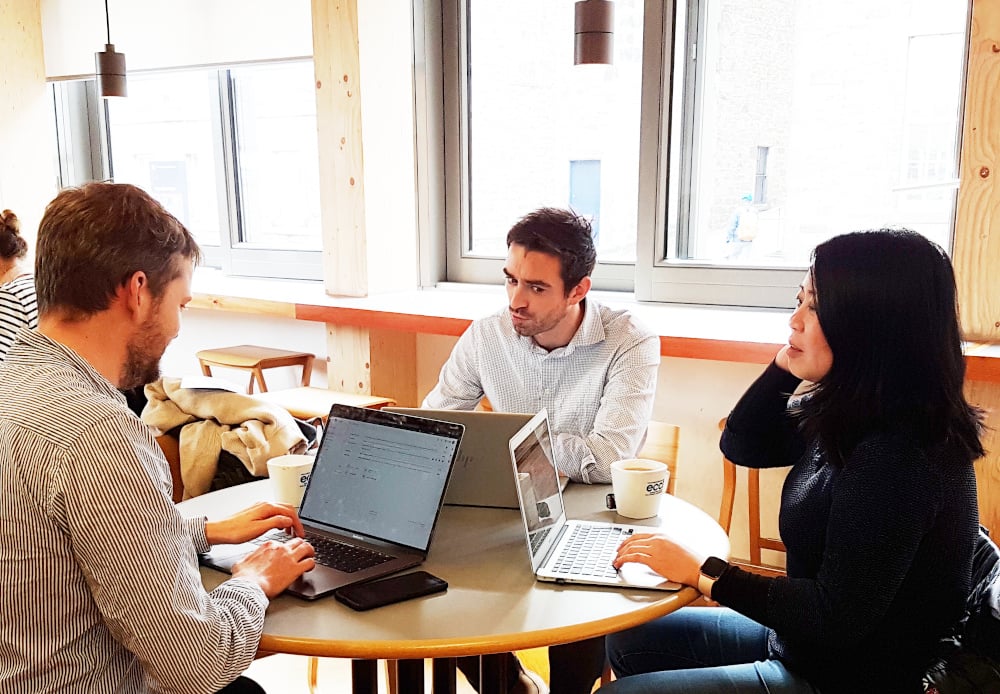In a cozy and modern coffee shop with bright, natural light streaming through large, sliding windows framed by unfinished wooden beams, three people are seated closely together at a small, round brown table. Each person is engrossed in their laptops, which are almost touching due to the table's size. They all have large coffee mugs in front of them. The woman on the right is Asian, with long dark hair, wearing a black sweater and dark blue jeans. To her left is a man with a beard, brown hair, and a black and white striped shirt. Opposite them sits another man with black hair, a mustache, and a five o'clock shadow, dressed in a light blue shirt. Behind them, window sills double as countertops with wooden stools neatly arranged underneath. Above each window-hovering over the scene-bookshelves and black pendant lights add to the modern aesthetic. The trio appears focused, perhaps collaborating or working individually, creating a serene and productive atmosphere.